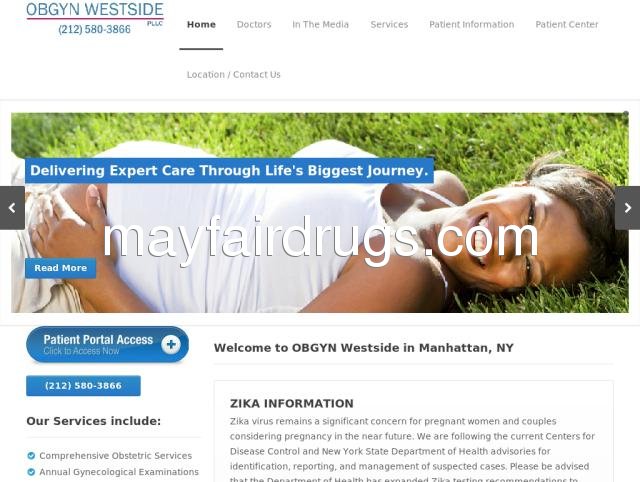A smiling pregnant woman, likely of mixed Mexican and/or Black heritage, reclines on a lush green lawn, facing the camera. Her brown hair is neatly tied back, highlighting her radiant smile and white teeth. She is wearing a white top with spaghetti straps, possibly a bathing suit or tank top, and a pair of shorts, though the lower part of her outfit is obscured by her baby bump. The photograph captures her joy and exudes a serene ambiance.

Adding to the scene, a blue banner with white text overlays the image, reading, "Delivering extra care through life's biggest journey." An arrow pointing left in white stands out on the gray left edge of the banner. Below the main caption, the website "mayfairdrugs.com" is displayed in small white letters, alongside a "Read More" button in blue with white text.

Positioned at the bottom of the image are additional interactive elements for users: a "Patient Portal Access" button with a plus sign, a button displaying a phone number, and information links labeled "Our services include" with various options available. A blue button with a check mark appears next to "Patient Portal Access," guiding visitors to more resources. Additionally, there's a welcome note from OBGYN Westside in Manhattan, New York, accompanied by information about Zika, presented in a detailed and informative manner.

Overall, the image and accompanying text combine to create a warm and welcoming introduction to maternal care services, delivered with a touch of personal connection and professional expertise.